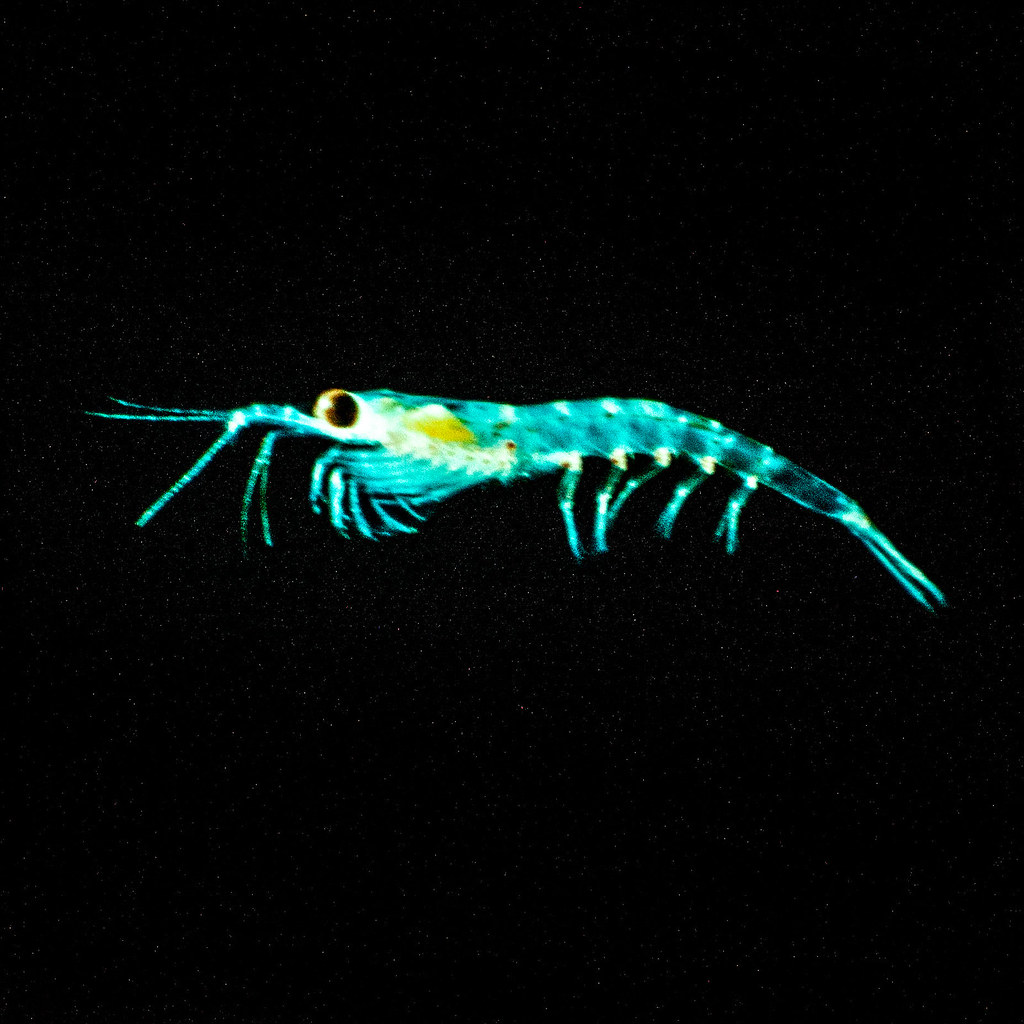The image showcases an enigmatic, bioluminescent sea creature set against a completely black background. Resembling a mix between a squid and a centipede, this neon blue, semi-translucent organism stands out brilliantly in the darkness. It features multiple legs and antennae, along with a prominent yellow or large black eye that pierces through the surrounding opaque void. The creature's slender, elongated body, which appears almost see-through, suggests it is an underwater entity, possibly captured through night vision or microscopic imaging, highlighting its intricate, glowing structure against the stark black backdrop.